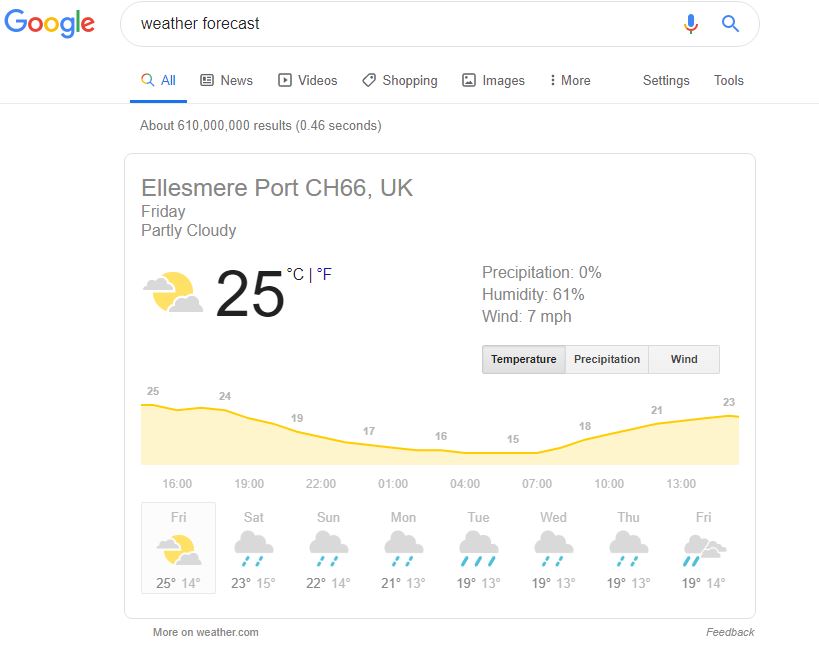This image appears to be a weather forecast card, likely sourced from a web application or a Google search result, for Ellesmere Port, CH66, in the United Kingdom. The main section of the card focuses on the weather for Friday, showing a partly cloudy day. A visual icon displays a yellow sun partially obscured by two white clouds, reinforcing the partly cloudy condition. Temperature readings show 25 degrees Fahrenheit (indicated by an "F" in purple).

The card provides additional meteorological data: 
- Precipitation: 0%
- Humidity: 61%
- Wind: 7 miles per hour

Below these details, there are three interactive tabs labeled "Temperature," "Precipitation," and "Wind." A line graph displays temperature fluctuations throughout the day, with time markers and corresponding temperatures. Starting at 4 PM (16:00) at 25°F, temperatures descend to 24°F by 7 PM (19:00), reach a low of 17°F by 1 AM (1:00), gradually rise to 16°F by 4 AM (4:00), and then climb back to 21°F by 1 PM (13:00). The temperature trend is depicted in yellow.

The bottom section features a weekly forecast, with Friday highlighted. Upcoming days include:
- Saturday: Cloudy with rain
- Sunday: Cloudy with rain

Similarly structured daily forecasts extend through the following Friday, providing a comprehensive overview of the week's weather patterns. Each day's forecast includes icons and temperature ranges, offering a user-friendly snapshot of future weather conditions.